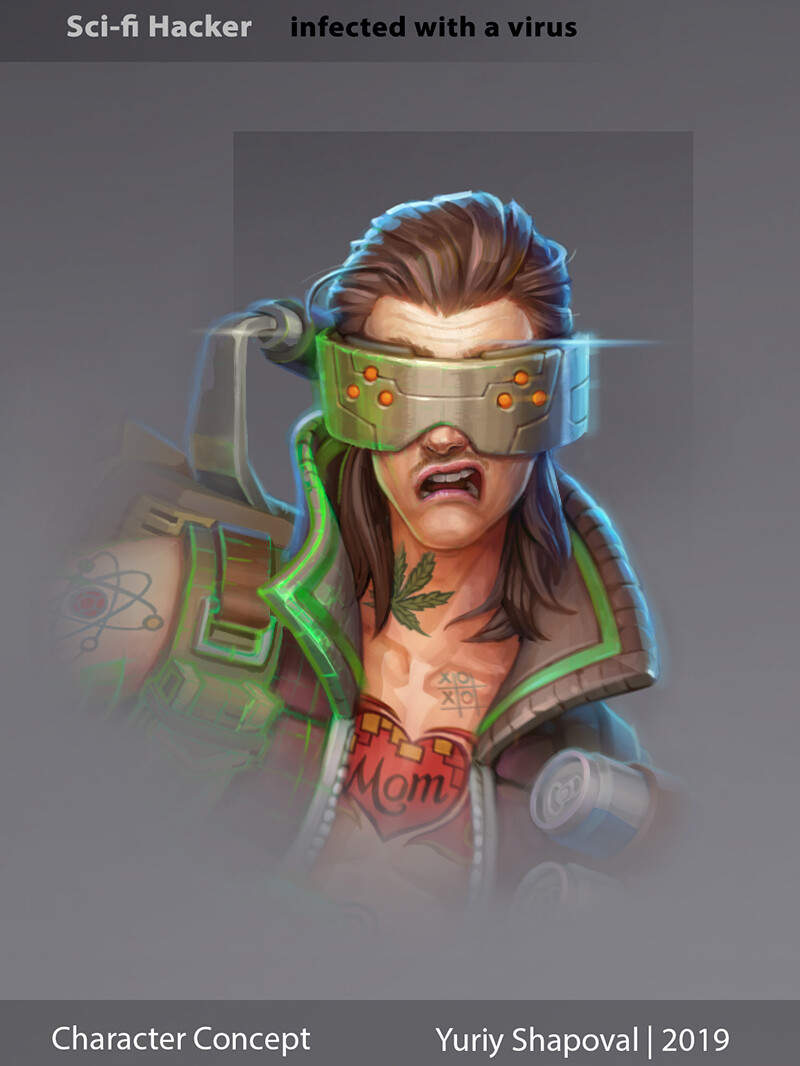This detailed character concept illustration features a "sci-fi hacker" labeled as "infected with a virus," set against a gray background with dark gray borders at the top and bottom. The top border transitions to a lighter gray on the right and includes the aforementioned text in white and black. The bottom banner, in white text, credits the concept to "Yuri Shapoval 2019."

The central figure of the illustration is a man depicted from the chest up. He sports long, slicked-back brown hair extending just past his shoulders. His facial expression is one of disgust, with his mouth open and downturned. He wears solid metal goggles, suggesting a futuristic or cybernetic function, and a distinctive brown, sleeveless, puffy vest. This vest features a green accent around the neckline and has beer cans strapped to the front.

His body is adorned with various tattoos: a green marijuana leaf on the right side of his neck (our left), a molecule on his right arm, a red heart on his chest that says "Mom," and a tic-tac-toe board above this heart on his left side. Adding to the sci-fi element, there is a metal attachment on his back.

Overall, the image is a detailed, character concept likely intended for a video game or comic book, expertly combining elements of sci-fi technology and a rebellious aesthetic.